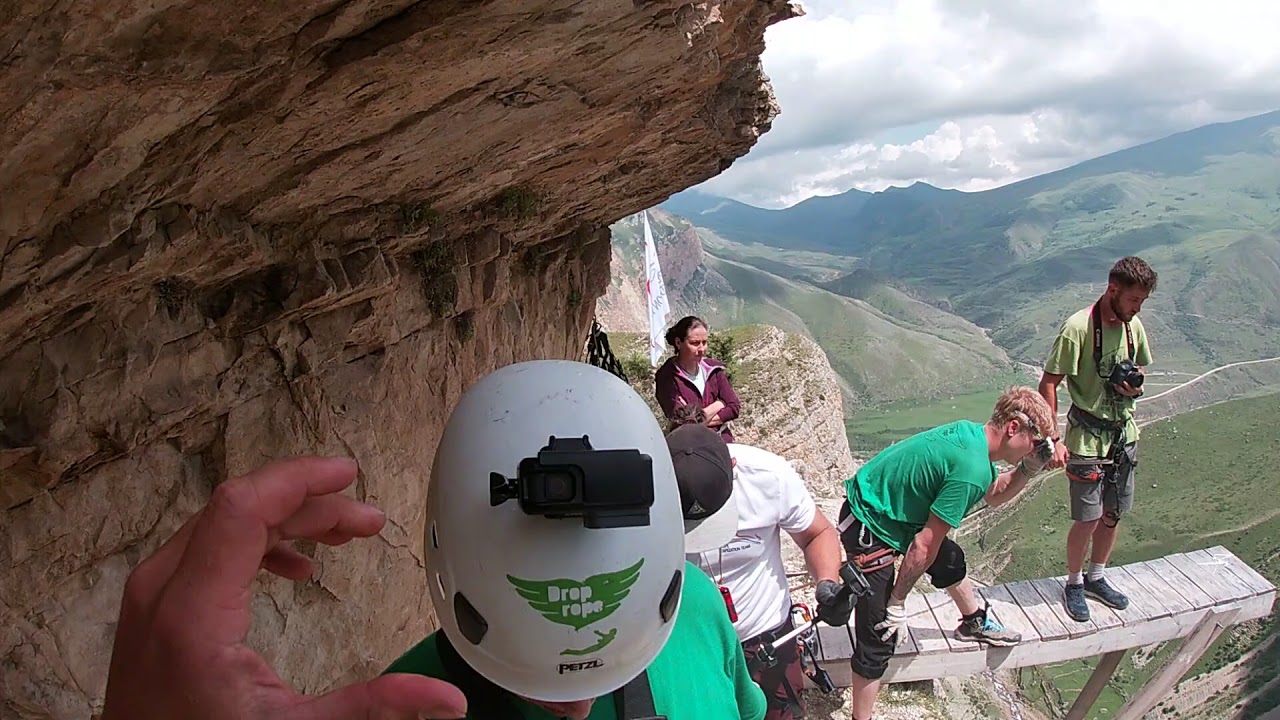In this highly detailed photograph, a group of five mountaineers stands on the edge of a rugged mountain cliff. The scene, viewed from a first-person perspective, showcases a diverse array of climbing gear and activities. To the left, the cliff's steep, brown rock formation dominates the frame, while the right side opens up to a lush, green valley filled with grass and trees, under a sky dotted with clouds.

A focal point is a wooden plank jutting out from the cliff, on which two men are precariously positioned. One man, equipped with a camera, gazes downward, possibly capturing the breathtaking view or planning his next move. Nearby, another man uses binoculars to scrutinize the terrain below. Both are engaged in their tasks, reflecting the adventurous spirit of the group.

In the foreground, a climber with a white helmet, marked by the words "Drop Rope" and decorated with a green wing-like logo, is seen reaching out, seemingly toward another person adjusting his helmet-mounted camera. The tension of the moment suggests that they are preparing for a challenging climb or a ziplining activity.

Standing slightly apart, a woman with her arms crossed observes the scene intently, perhaps assessing the situation or waiting for her turn. Her contemplative stance adds a sense of calm amid the group's high-energy preparation. The background reveals a sweeping view of towering mountains and a verdant valley below, highlighting the dizzying height and the expansive natural beauty surrounding them.